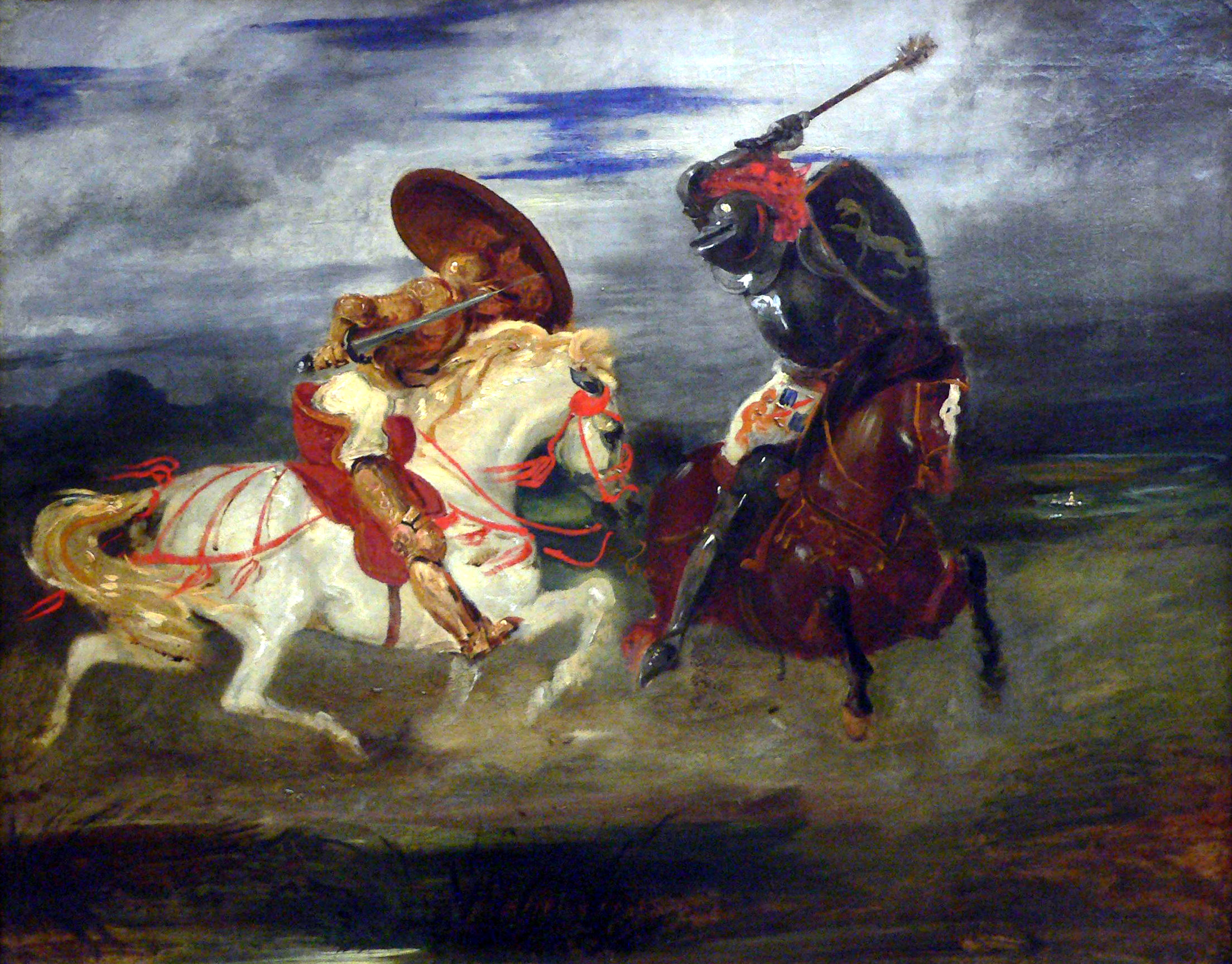In this dynamic detail of an oil painting, two warriors are locked in fierce combat on horseback against a dramatic backdrop. Charging in from the left, a white horse adorned with red saddlery and ornate red tassels flies through the air, with its brownish tail streaming behind. The rider, clad in gleaming gold armor, is poised with a sword in their right hand and a shield lifted high in their left, ready to strike or defend as necessary.

On the right, a sturdy chestnut horse stands resilient, its black lower legs and dark mane adding to its imposing presence. Its rider is fully armored in black and dark gray, accented with touches of red. The black-clad warrior brandishes a formidable weapon, likely a club or a mace, held aloft to counter the sword-wielding adversary. Their shield, bearing an animal insignia, possibly a lion or tiger, reflects their readiness for combat.

Set against a turbulent sky of gray and white with hints of blue, and grounded on a dark, earthy landscape with patches of dark brownish-green, the scene exudes tension and drama. Mountains loom in the distance, and the cloud-filled sky heightens the atmosphere of an intense battlefield encounter.